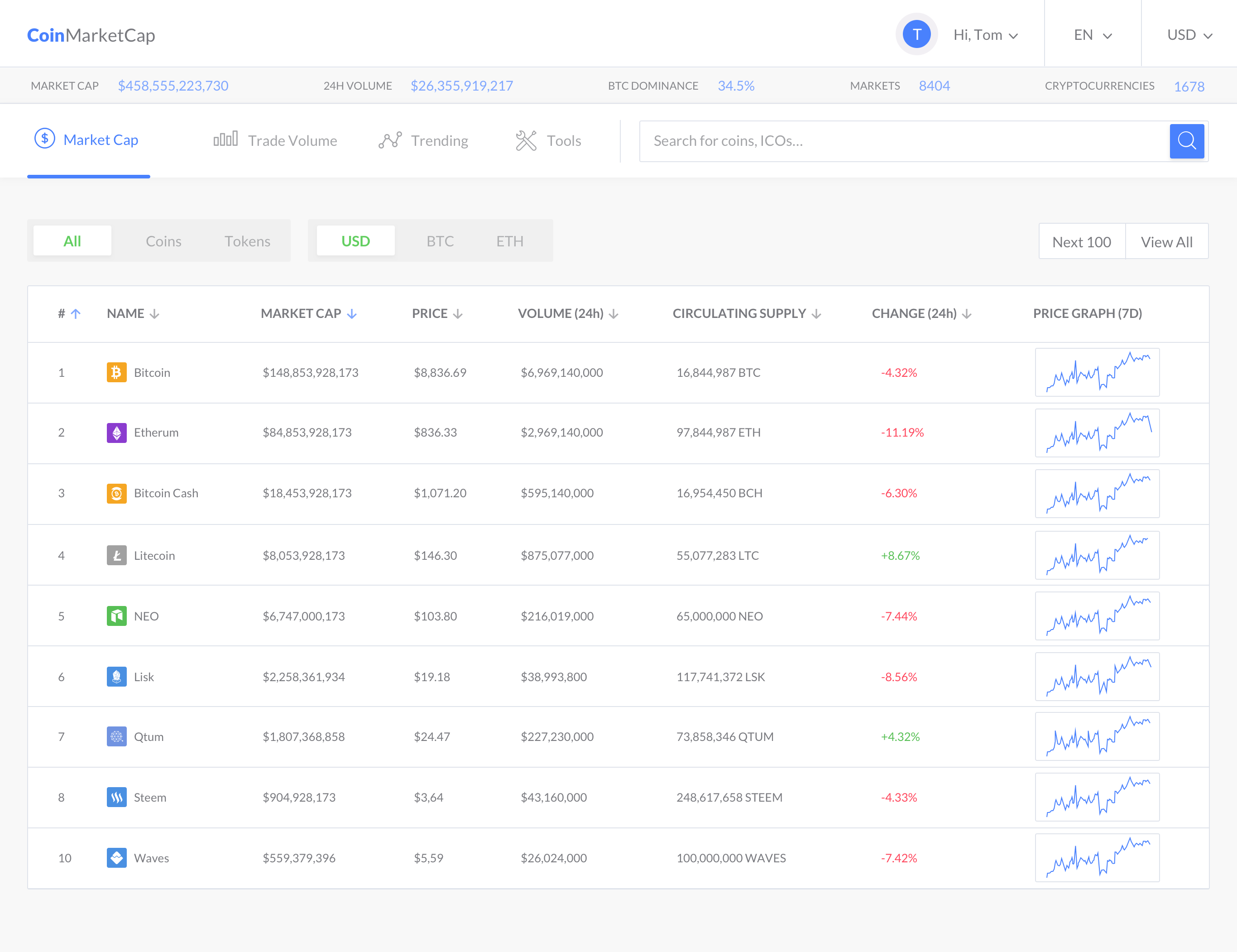The image features a light blue background with a prominent header at the top that reads "CoinMarketCap". Adjacent to the header are several interactive elements: a blue circular button with a white "T" inside, labeled "Hi, Tom" followed by a down arrow, an "EN" button with a down arrow indicating language selection, and a "USD" button with a down arrow for currency selection.

Below these buttons, there is a blue box displaying important financial metrics in hard-to-read blue text – these metrics include "Market Cap," "24 Hour Volume," and "BTC Dominance." Beneath this blue box, there is a larger white area. At the top of this white section, "Market Cap" is underlined in blue, followed by headers for "Trade Volume," "Trending Tools," and a search function for coins. There is also an "ICOs" section and a small blue box featuring a magnifying glass icon, which serves as a search button.

Further down, another interactive section contains buttons labeled "All Coins," "Tokens," "USD," "BTC," and "ETH," along with two additional buttons for "Next 100" and "View All."

Immediately below, the background remains white but now features ten numbered boxes in a list format. Each box includes various columns marked with an up arrow or down arrow such as "Star," "Name," "Market Cap," "Price," "Volume 24 Hours," "Circulating Supply," "Change 24 Hours," and a "Price Graph." The shaded bars in these columns are color-coded: orange for the first, purple for the second, followed by a succession of orange, gray, green, and different shades of blue.

Next to the price graph metric are numerical changes in percentages like -432%, -1119%, -6.3%, +8.67%, -744%, -6.56%, +4.32%, -4.3%, and +6.4%. Lastly, blue graphical trend lines are seen on the far right of each row.